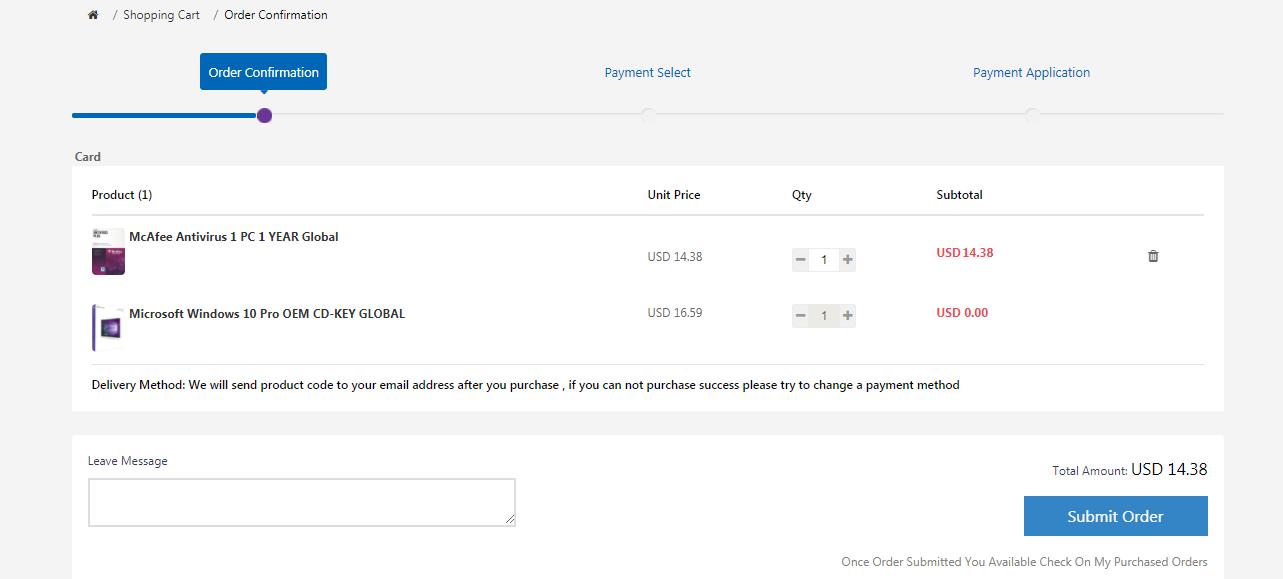The image depicts an online shopping cart interface with detailed elements related to the purchase process. In the top left corner, an icon of a house is displayed. Next to it, there's a shopping cart icon followed by a blue rectangle labeled "Order Confirmation." Below, various sections are outlined including "Payment Select" and "Payment Application," specifically featuring a "Texas card" option.

The product list includes:
1. McAfee Antivirus: One PC, one year global license for USD 14.38. Quantity adjustment buttons (gray minus and gray plus) are present, as well as a trash can icon.
2. Microsoft Windows 10 Pro OEM CDK global: Listed price is USD 16.59, but it shows minus one plus with a subtotal of USD 0. 

For the delivery method, the instructions state that the product code will be sent to the customer's email address after the purchase. If the purchase is unsuccessful, customers are advised to attempt a different method. An option to "Leave a Message" is mentioned.

At the bottom, the total amount is listed as USD 14.38. A blue rectangle button labeled "Submit Order" is visible, with text underneath indicating that once the order is submitted, customers can check their purchased orders. Lastly, a gray "Backwards" button is shown, highlighted multiple times as "gray, gray, gray."

The overall interface is a shopping cart for purchasing antivirus software and a Windows operating system.